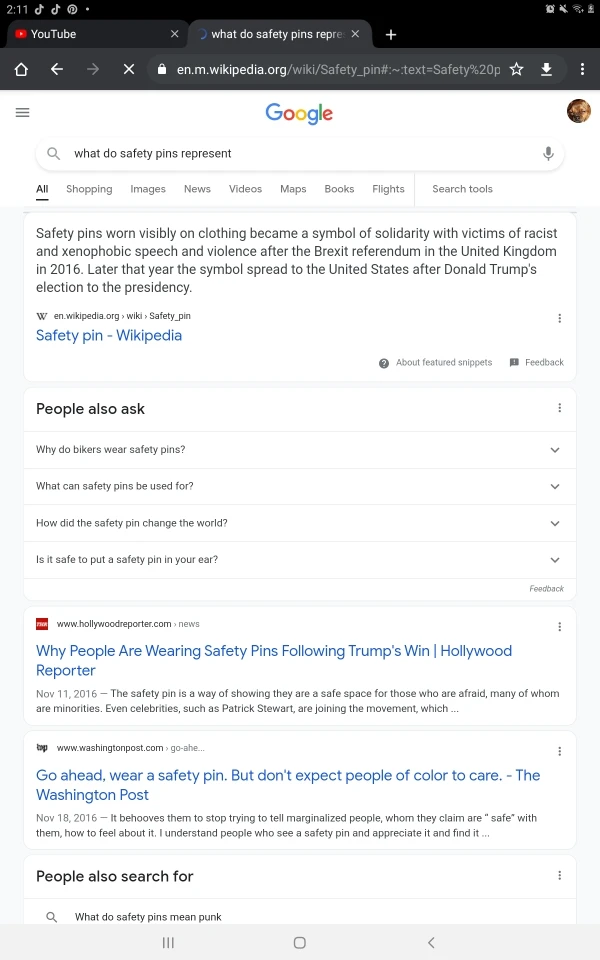Here is the cleaned-up and descriptive caption:

---

Screenshot of a Google search for "why do safety pins represent." The search results explain that safety pins, often visibly worn on clothing, symbolize solidarity with victims of racism. The "People also ask" section includes related queries such as "why people are wearing safety pins" and "following." One search suggestion reads, "go ahead, wear a safety pin, don't expect people of color to care." The screenshot also shows the user's open YouTube and TikTok tabs, a profile picture in the top right corner, and a black top navigation bar.